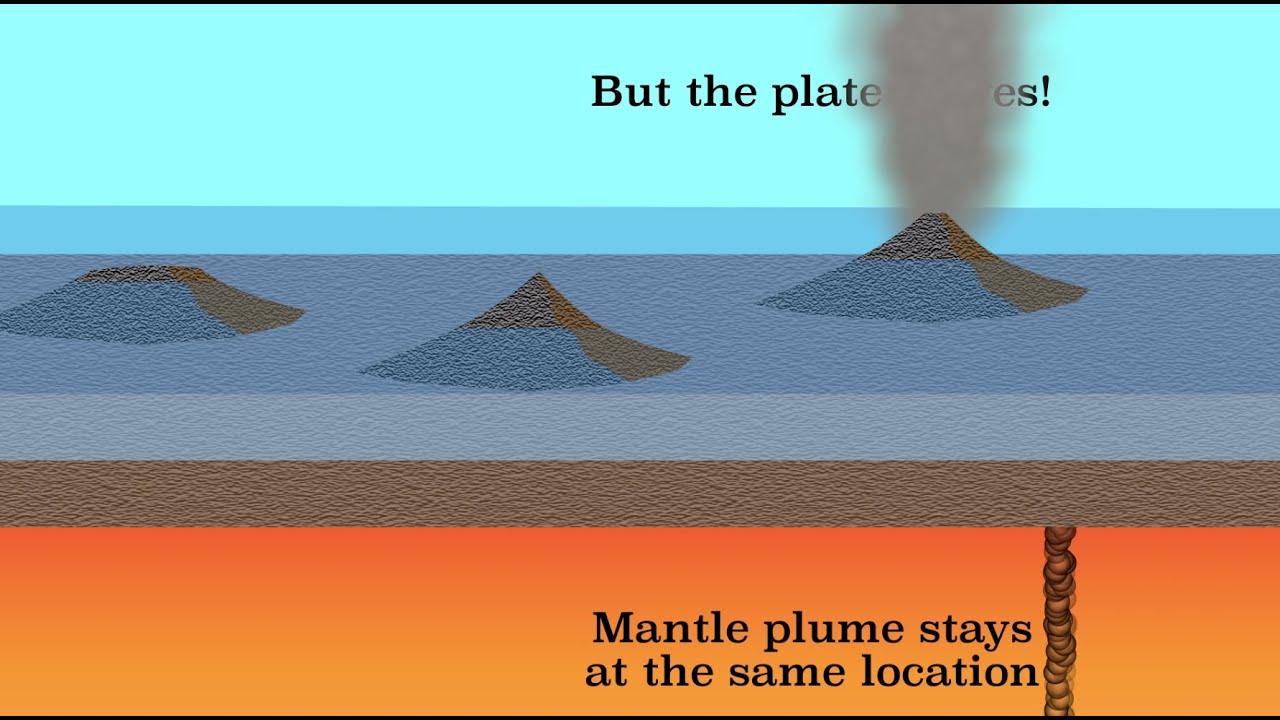The image depicts the formation of the Hawaiian Islands through volcanic activity. At the bottom, a mantle plume in vivid red and orange colors illustrates the upwelling of molten lava from beneath the Earth's crust. Above the mantle, a brown layer signifies the ground or oceanic crust, topped by a transparent blue layer suggesting the ocean. Rising through these layers are three volcanic islands. From left to right, the islands decrease in age, with the rightmost island showcasing an active volcano, spewing ash and smoke into the sky, partially obscuring a sentence that seems to read "but the plate moves on," ending with an exclamation mark. This image graphically demonstrates how the stationary mantle plume continuously forms new islands as the tectonic plate moves over it, leaving older, eroded islands further to the north. The intricate details highlight the fascinating geological process responsible for creating the Hawaiian archipelago.